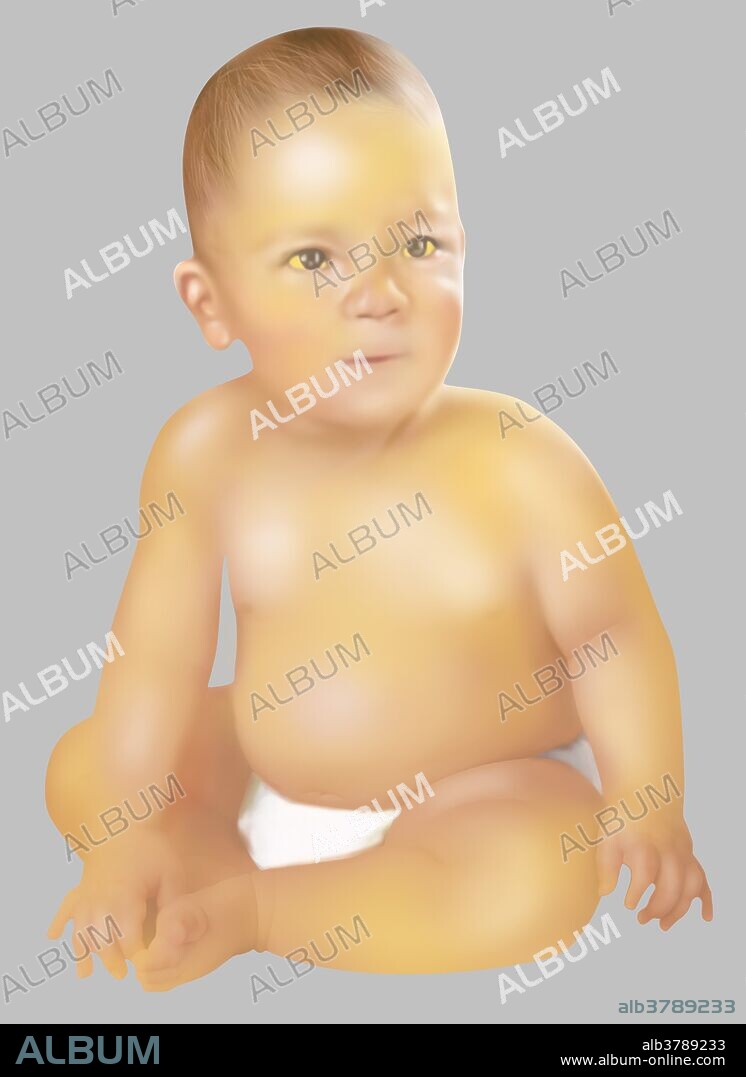This digitally rendered image features a plump Caucasian male infant, appearing only a few months old, sitting with legs crossed and wearing a white diaper. The baby's skin has a yellowish tone, potentially giving a jaundiced appearance, with yellow tints noticeable on the eyelids and the whites of the eyes which are unusually black. The baby, adorned with a half-smile, is placed against a gray background. The word "ALBUM" appears diagonally across the image in alternating white and gray text. At the bottom, there is a black strip featuring the text "ALB3789233" and the website "www.albumonline.com." The image gives the impression of being a stock photo or test graphic, prominently displaying branding elements and company information.